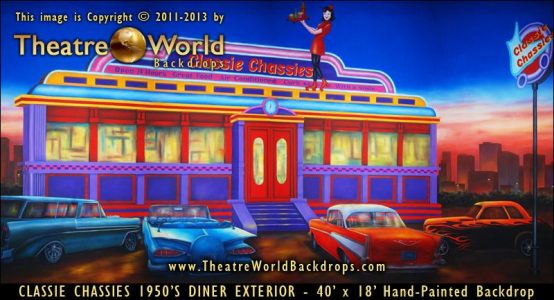This vibrant painting depicts a lively 1950s-style diner scene, likely intended as a promotional poster or backdrop. The diner, named "Classic Chassis," features bright neon lights in turquoise and pink, with red-framed front windows and double doors accessible via purple stairs. A notable detail is the statue or mannequin of a roller-skating waitress in a red uniform, black pants, and red skates, perched atop the roof and holding a tray. 

In front of the diner, there are several vintage cars, including a red and white '55 Chevy, a striking hot rod with orange flames on black paint, a turquoise blue vehicle, and another orange car. They evoke the era's iconic automotive style with fins resembling rockets. The background showcases a city skyline with a dark reddish-blue sky, accentuating the nostalgic mood.

Signage includes golden text reading "Theater World" with a planet illustration, and a circular neon sign on a pole in the parking lot saying "Classic Chassis." The image is credited to Theater World Backdrops, with a copyright from 2011 to 2013, and includes their website, www.theaterworldbackdrops.com. The dimensions of the hand-painted backdrop are noted as 40 feet by 18 feet.